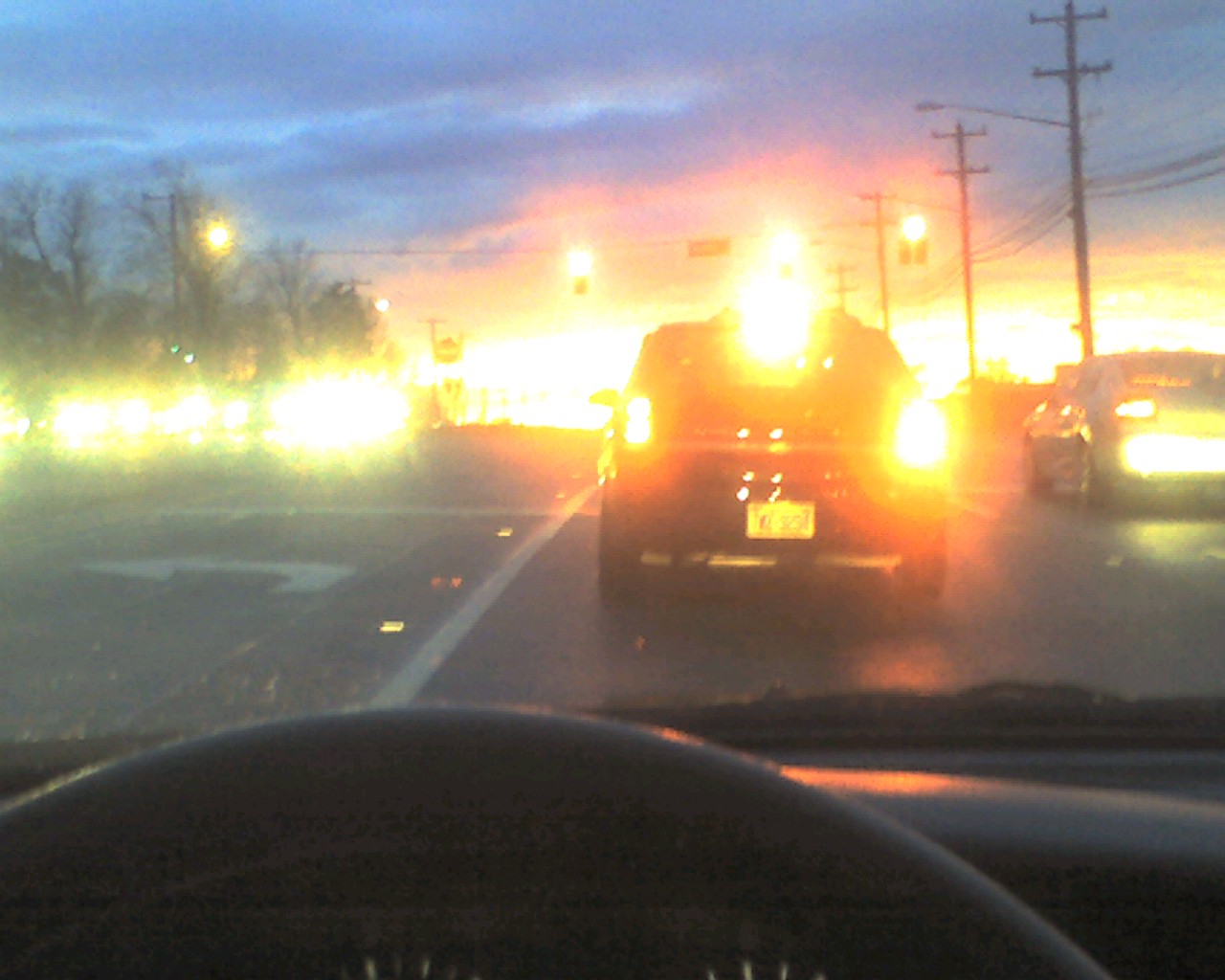Caption:
A captivating evening photograph taken from the inside of a car from the driver's side perspective. The image, shot through the front windshield, showcases the black top of the steering wheel and the black dashboard silhouetted against the evening glow. Two lanes of oncoming traffic are visible on the opposite side of the street, while the driver follows a black car, indistinct yet bathed in the soft glow of streetlights and headlights. The sky, a dramatic display of purplish-red hues mingled with dark gray-blue clouds, reflects the onset of twilight, creating a serene and atmospheric scene.